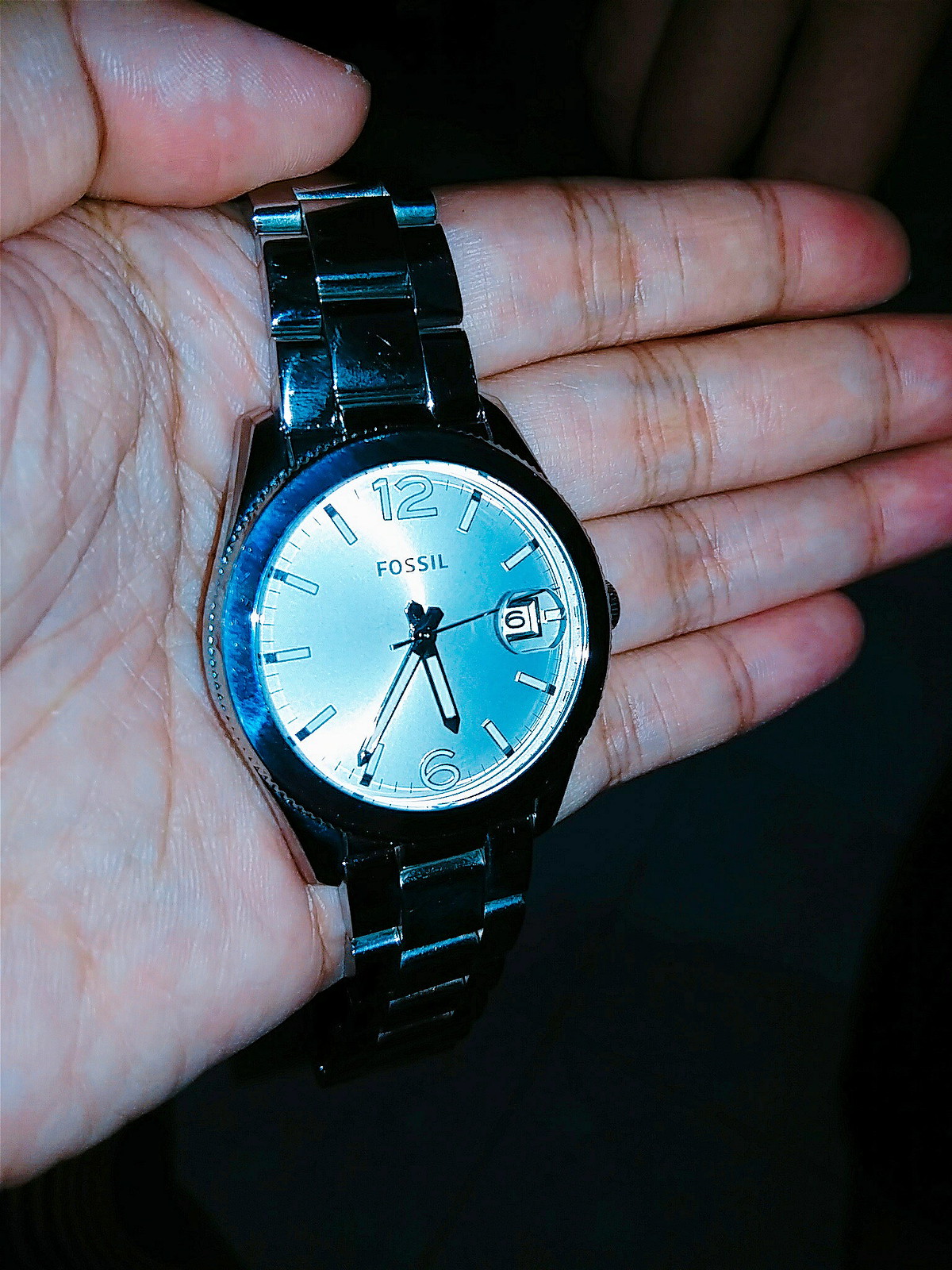In this close-up photograph, a metal wristwatch branded "FOSSIL" is prominently displayed, held delicately in a hand rather than worn on the wrist. The watch's band envelops the individual's four fingers, with the thumb slightly overlapping the top edge. The timepiece gleams with a polished, silver-colored dial, showcasing the brand name "FOSSIL" in a contrasting dark gray. The functional design is evident as the small hand indicates a time just past the five, while the large hand is slightly beyond the seven, suggesting the time reads approximately 5:36. This detailed shot captures the watch's intricate craftsmanship and elegant detailing.